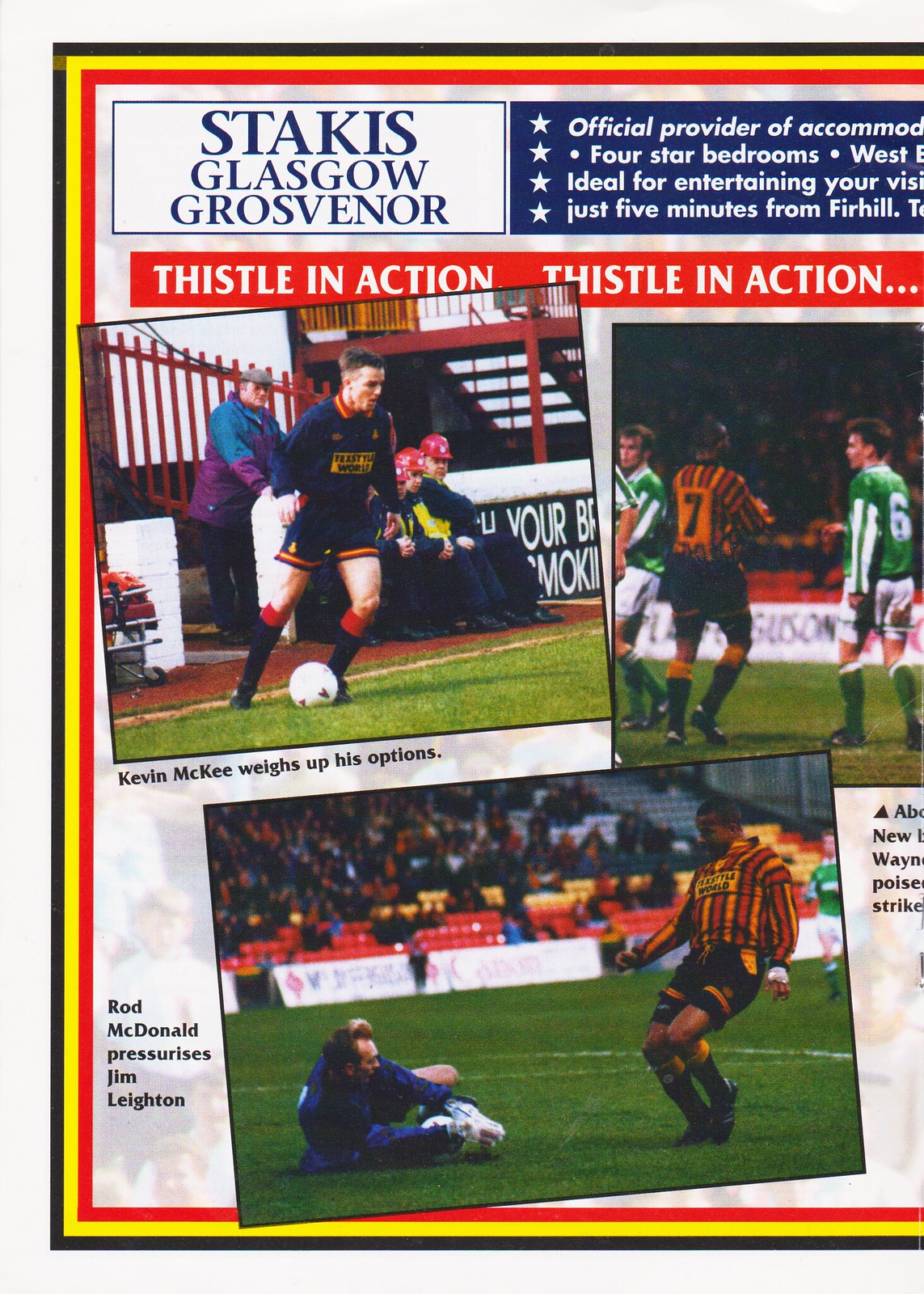The image appears to be a partial poster or magazine page advertising for the "Stakis Glasgow Grosvenor" with a predominantly white background edged with black, yellow, and red lines. In the top left corner, the text "Stakis Glasgow Grosvenor" is prominently displayed in blue letters. To the right, there is a blue box with white text and star-shaped bullet points, some of which are cut off. It partially reads: "official provider of accommodation," "four-star bedrooms," and "ideal for entertaining your visit, just five minutes from Fir Hill." Below this text, in a red strip with white letters, the phrase "Thistle in Action, Thistle in Action" is repeated.

The poster features three distinct photographs of soccer players in action. The top left photograph, captioned "Kevin McKee weighs up his options," shows Kevin McKee in a dark blue long-sleeved jersey with an orange collar, dark blue shorts with an orange trim, and blue socks with red tops, standing poised with a white soccer ball. To the right of this image is another photograph of a soccer scene, though its caption is not fully visible. The bottom photograph, captioned "Rod McDonald pressurizes Jim Layton," depicts Rod McDonald in a vertically striped orange, red, and black shirt in an intense moment of gameplay. The background features silver bleachers filled with spectators and various signs partly obscured by the action on the field.